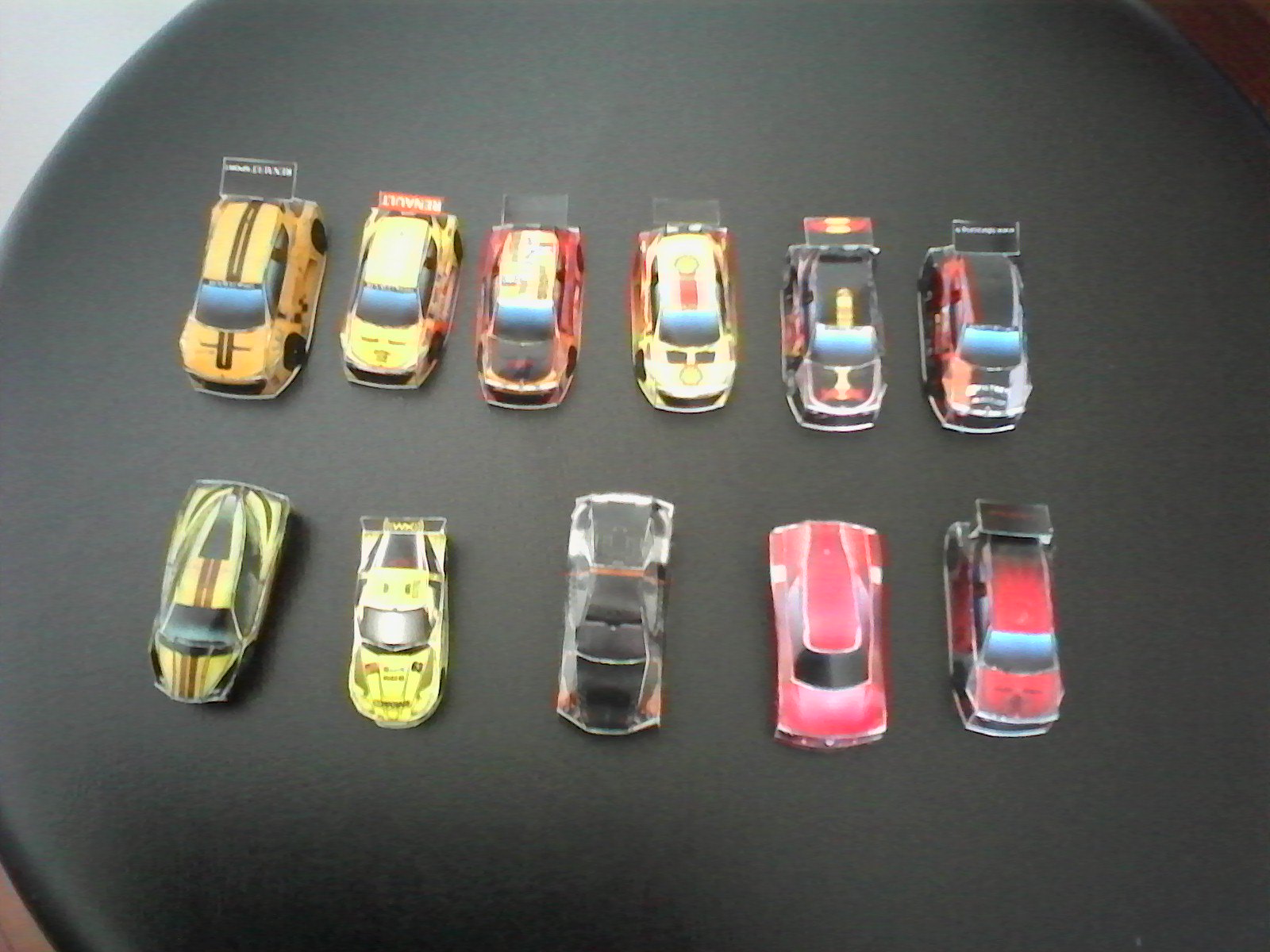The image is a grainy, slightly out-of-focus photo of 11 die-cast toy cars, possibly Hot Wheels or Matchbox cars, arranged in two rows on a round, black, leathery surface, likely a tabletop or barstool. The top row consists of six cars positioned side by side, and the bottom row contains five cars. The cars are viewed from above, revealing their varied colors and designs. Predominantly, the cars in both rows are yellow and black, with some featuring stripes. There's also an orange car with black stripes, a couple of red cars, and one pink, futuristic-looking vehicle. While most cars in the top row have spoilers, one car in the bottom row also features a spoiler. The vehicles appear well-organized, though the criteria for their arrangement are unclear.